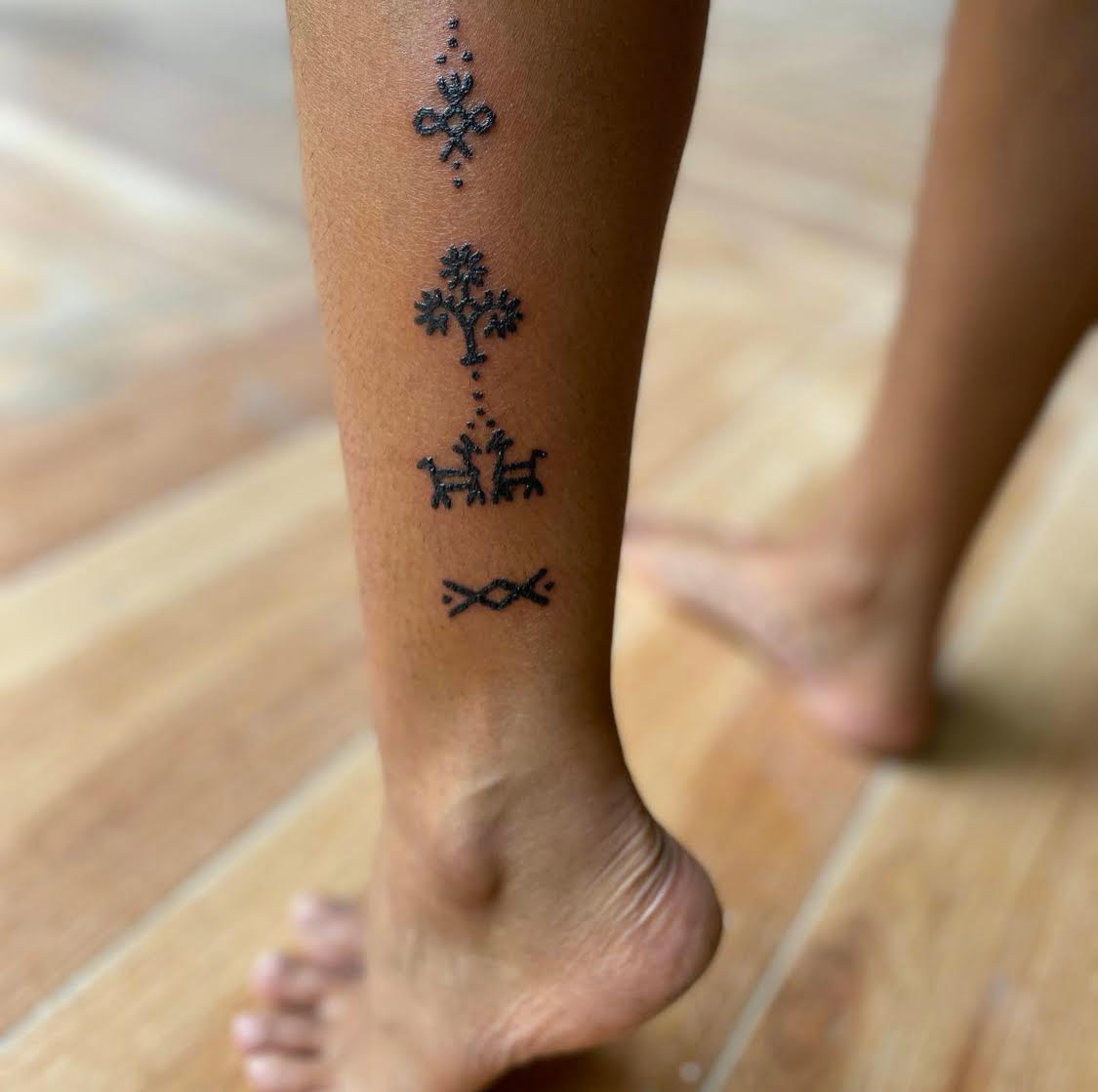The image shows the back of a woman's calves on a wood-grain floor that appears to be cedar-like with a tan grout. The woman has a dark complexion and is standing on her tippy toes on her left foot, with the right foot flat on the ground. The focus is on her left calf, which features a series of four distinct tattoos running vertically:

1. At the top, there's a symbol comprised of three dots forming a triangular crest, topped with three lines, and an X shape beneath it.
2. Below that, a tattoo depicts a stylized tree with branching circles, flanked by dots, leading down to two small stick-figure deer facing each other.
3. Further down, there's a tattoo resembling two overlapping X's with dots in the spaces between the arms.
This intricate and symbolic tattoo sequence is accentuated against her tan skin, creating a striking contrast with the wood-grain floor beneath her.